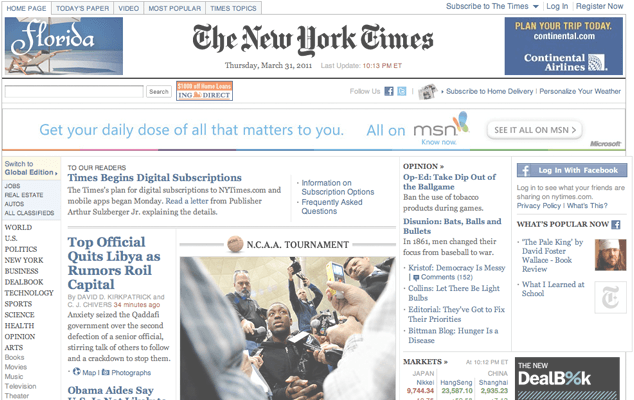The image depicts the homepage of The New York Times online, showcasing its features and structure as it appeared on Thursday, March 31, 2011. At the top left, there is a navigation menu including options like 'Home Page', 'Today's Paper', 'Video', 'Most Popular', and 'Times Topics'. On the right side, also starting from the left, there are options to 'Subscribe to The Times' with a dropdown menu, 'Log In', and 'Register Now'.

Underneath this, a section on the left announces 'Florida' in white text over a photo of a beach scene. Dominating the center, the header 'The New York Times' is displayed in the largest font, followed by the date 'Thursday, March 31, 2011,' and a timestamp 'Last updated: 10:13 PM Eastern Time' in red text.

On the right side, an advertisement prompts users to 'Plan your trip today at continental.com' for Continental Airlines. Below this advert is a thin black line followed by a search bar. Further down, another promotion reads 'Get your daily dose of what matters to you, all on MSN. See it all on MSN.'

The main content area is divided into various sections with headlines such as 'To Our Readers: Times Begins Digital Subscriptions,' 'Top Official Quits Libya as Rumors Roil,' 'Capital,' and 'NCAA Tournament.' The 'Opinions' section features an op-ed titled 'Take Drip Out of the Ballgame,' a discussion labeled 'Bats, Balls, and Bulletins,' an article named 'Race for Democracy Is Messy' with 152 comments, and a piece titled 'Collins: Let There Be Light Bulbs.' The 'Editorial' headline reads 'They're Not.'

This detailed layout provides a snapshot of the website’s structure, articles, promotional content, and available features as of the specified date and time.